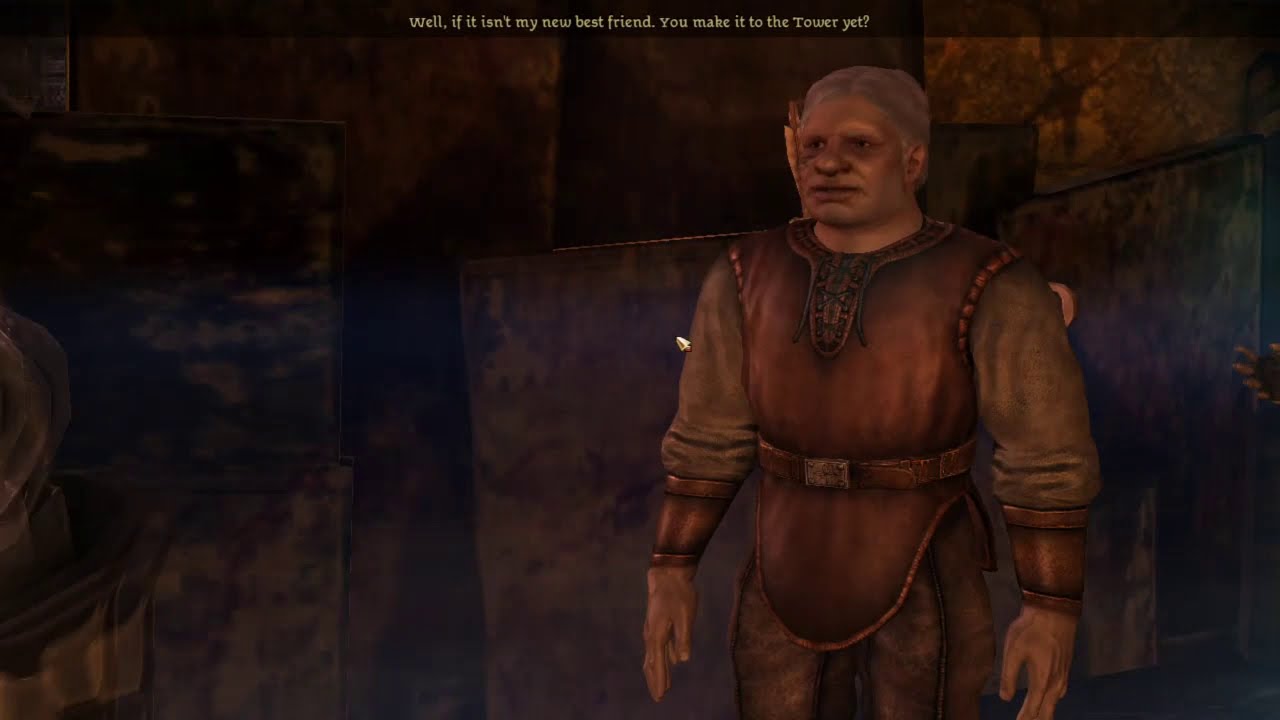The image is an animated screenshot from a video game or a cartoon, displaying a rather dimly lit scene that's predominantly brown and copper in hue. The background features a rock or stone wall, giving an impression of either an indoor medieval setting or a labyrinthine structure. Dominating the right-hand side of the screen is a male character who closely resembles Varric from Dragon Age, hinting that he might be a dwarf. He is dressed in a rust-brown medieval-style tunic adorned with intricate designs at the neck, layered over a brown shirt. His attire includes a belt with a gold clasp, gold cuffs or possibly bronze arm guards, and dark pants. The character has short, possibly gray hair, and a wide, flat face, oriented towards the left side of the screen, though what he's looking at isn’t visible. At the very top of the screen, over a transparent black bar, there's white text that reads, "Well, if it isn't my new best friend, you make it to the tower yet?"